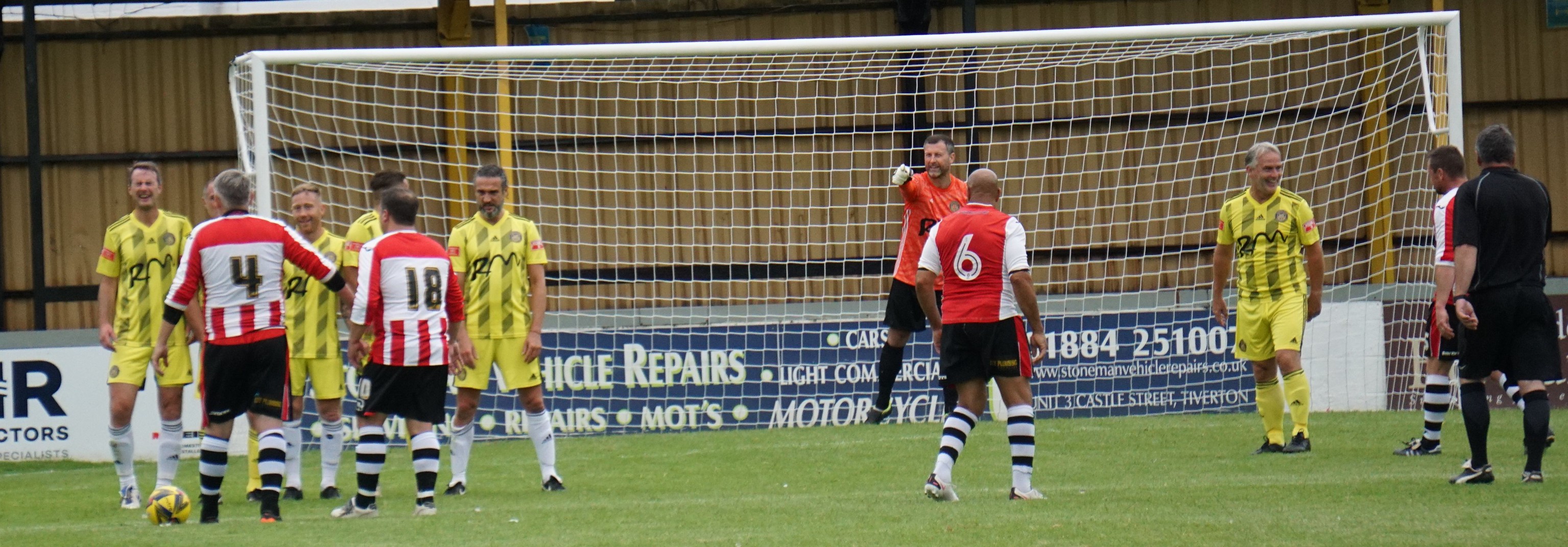This photograph captures an intense moment before the start of a soccer game between two teams of older male players, possibly in their 50s. The teams are distinctly dressed, with one team wearing orange and white, and the other in yellow and green. The scene is set on a green field, with the goalposts and net prominently visible in the background. Behind the goal, there's a long blue banner featuring advertisements related to vehicle repairs or motorcycles.

In the foreground, five players from the yellow and green team are positioned in front of the goal along with two players from the orange and white team, who have their backs to us, displaying the numbers 4 and 18 on their jerseys. The atmosphere suggests they are preparing for a penalty kick, as they are not in motion but rather aligning strategically.

To the extreme right, a referee dressed in all black can be seen, possibly giving instructions or ensuring fair play. The orange and white team's goalie is also in the shot, positioned in front of the goal and pointing, likely directing his teammates. The photo is taken during the daytime, in a wide format that captures a panoramic view of the players, the field, and the advertisements in the background.